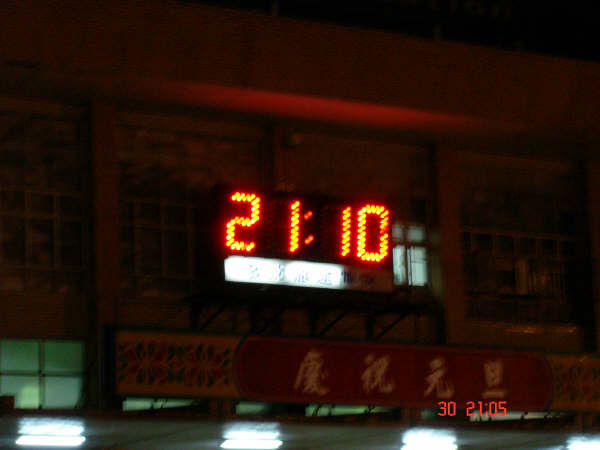The image features a prominently lit digital clock displaying military time, reading 21:10 in bright red-orange numbers. The clock, which stands out against the dark evening setting, is attached to a sign adorned with Southeast Asian writing, possibly Cambodian, rather than Chinese characters. Below this time display, there's additional text and intricate decorative flower designs on the signage. The scene appears to take place in an outdoor market or street in an urban area, characterized by the surrounding taller buildings in the background. The signage also includes a series of images depicting various outdoor activities, though the nighttime lighting makes the specific details challenging to discern. The clock’s light partially illuminates its surroundings, revealing structural beams and the outlined shapes of four-pane windows below. Interestingly, while the clock displays 21:10, the photograph’s metadata indicates a capture time of 21:05, creating a small discrepancy.